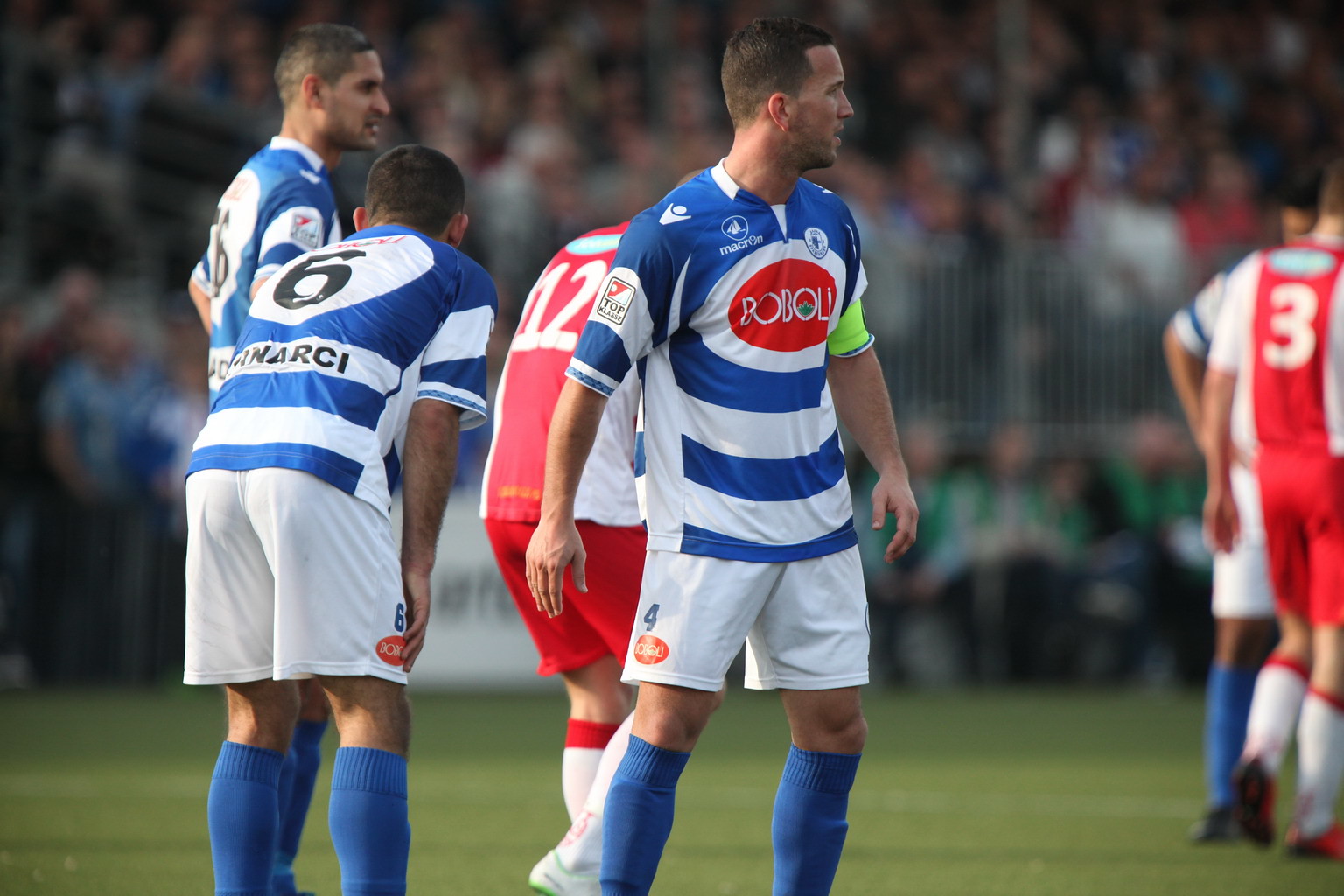This outdoor photograph captures the intensity of a soccer match taking place on a lush green field, likely in the middle of the day. Central to the image is a soccer player, or footballer, wearing a blue and white striped jersey with white shorts and blue socks, glancing off into the distance to the right. His jersey reads "ROBOLO" in white letters against a red background, and his shorts display the number 4. 

Behind him, to the right, stands another player in a red and white uniform, with the number 12 clearly visible on his back as he is turned away. To the left, another player in a blue and white uniform, numbered 6, is also facing away, with the number visible both on his back and shorts. Obscured by this player is another teammate, also clad in blue and white and looking right. On the far right of the image, two more players are discernible—one in a red and white uniform with the number 3, and another mostly hidden but similarly dressed in blue and white.

The background reveals blurred spectators in the stands, enhancing the atmosphere of the engaged crowd watching the game. Although slightly out of focus, the fans add a sense of excitement and immersion to the scene. The picture is composed with a variety of colors, noting green, blue, tan, white, red, gray, and brown, emphasizing the dynamic and vibrant setting of this live soccer match.